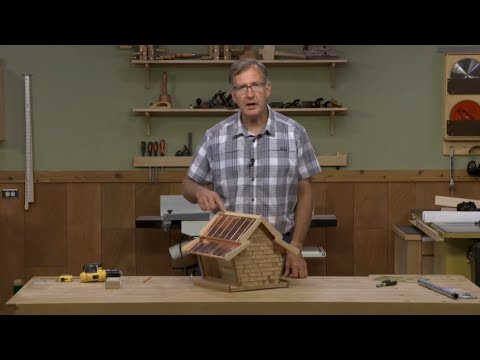In this indoor photographic image, a middle-aged white man with gray hair cut short and wearing glasses stands behind a light brown woodworking table. He is dressed in a short-sleeved, gray and white plaid, button-down collared shirt, to which a microphone is attached. He appears to be staring directly into the camera with a slightly surprised expression. The table before him is organized with various tools, including a yellow and black power drill on the left and a silver rod, potentially a level, on the right. Centrally placed on the table is a meticulously crafted wooden birdhouse with gabled roofs and glass panes. To the right of the table rests a pipe. The setting is detailed with a backdrop featuring a green wall with wooden wainscoting halfway up. This backdrop includes several shelves displaying numerous woodworking instruments such as planes, chisels, and saw blades mounted on the wall. Additionally, another workbench or possibly a power saw can be observed to the right. The photograph itself is horizontally aligned and framed with a thick black border at the top and bottom, capturing a vivid and detailed scene of the man's recent craft project and his well-equipped workshop.